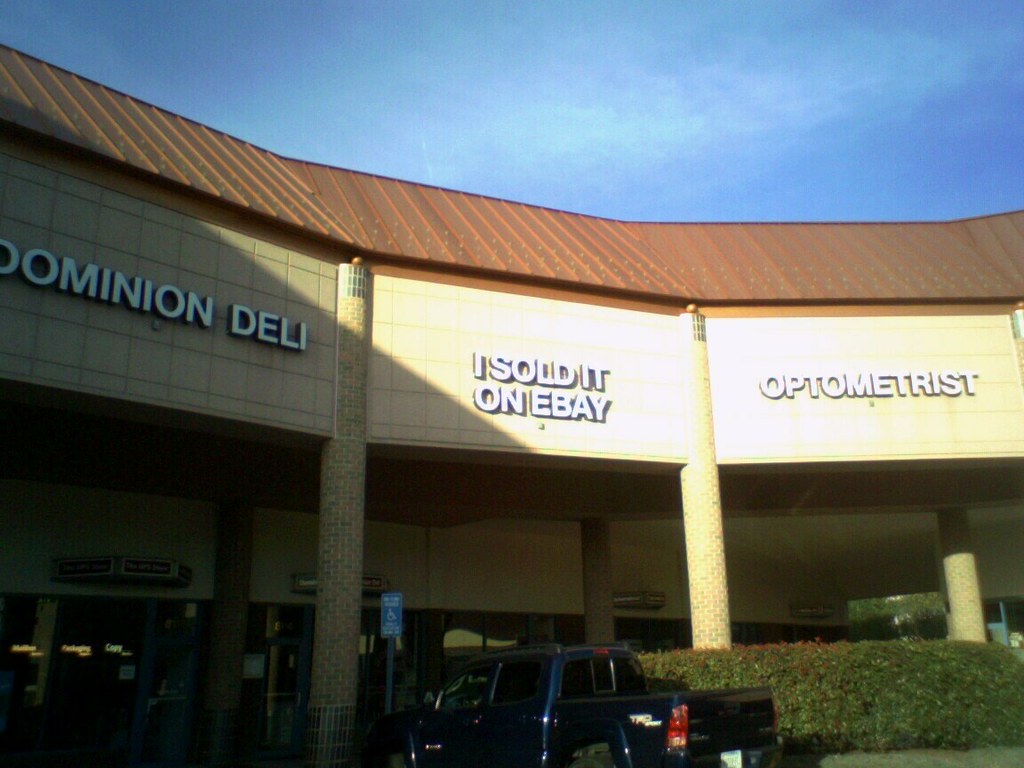This photograph captures the exterior of a tan-colored storefront building with distinctive architectural features and three different businesses. The building is adorned with lighter-colored brick stone pillars that vertically segment rectangular portions of a tan-tiled wall. Above, a slanted roof in a reddish-brown hue adds a striking contrast to the structure. Bright sunlight illuminates the two right rectangular panels, leaving the far-left panel in shade, under a vibrant blue sky.

In front of the building, a navy-blue pickup truck is parked in a designated handicap spot, marked by a clearly visible blue and white handicap sign. The storefronts feature three different business signs: the far-left rectangle displays "Dominion Deli," the middle one advertises "I Sold It on eBay," and the far-right panel reads "Optometrist." The glass storefront windows enhance the welcoming appearance of the building, reflecting the clear day outside.